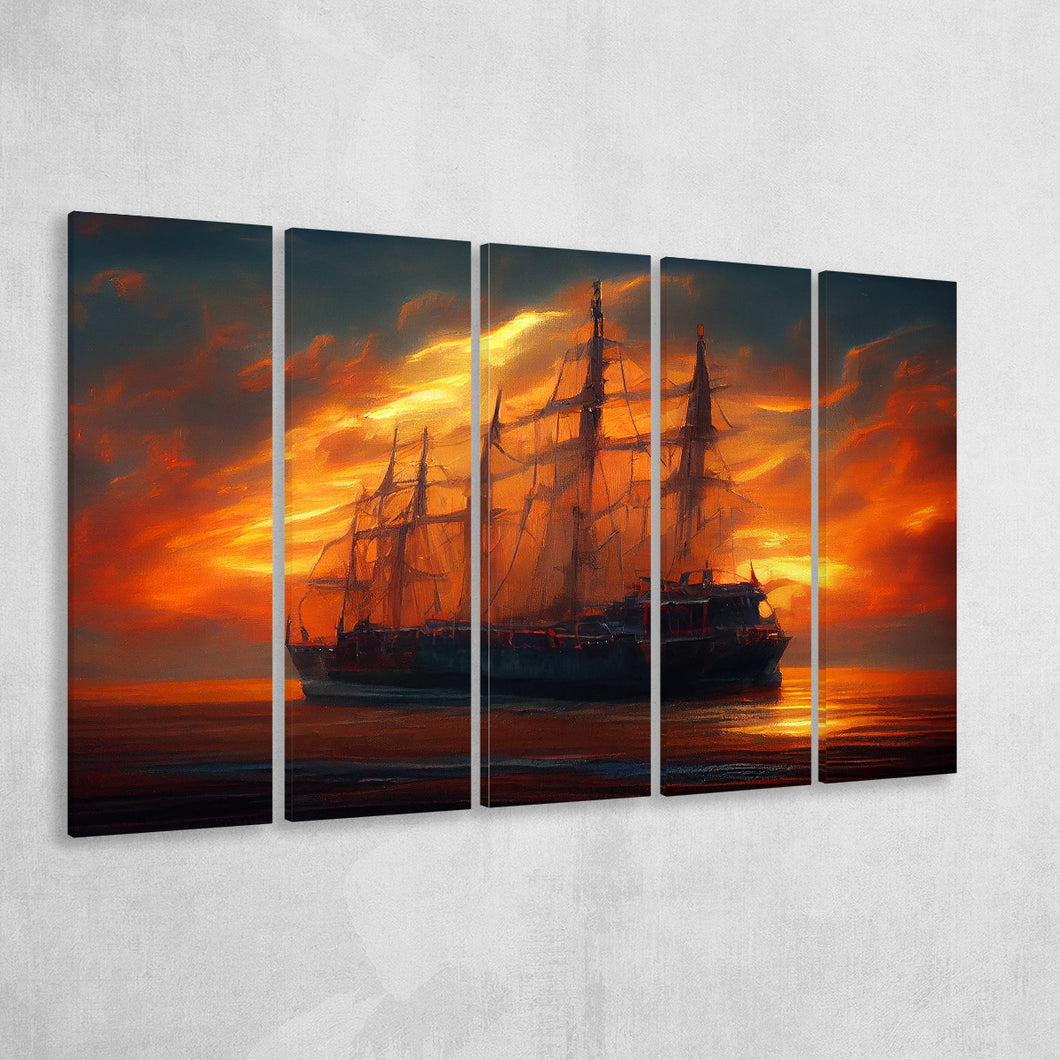This image showcases a highly detailed digital rendering of an expansive oil painting split into five separate canvas pieces. Mounted against a backdrop of textured cement or marble-colored wall, each canvas collectively forms the entirety of a striking maritime scene. The artwork depicts a large, old naval ship with massive masts and sails, set against a fiery sunset. The upper portion of the scene features a dark, almost black sky transitioning into blazing hues of yellow, orange, and dark red flames. The ship, which exudes a dark and grungy aesthetic, sails on the sea beneath the sunset, with the water reflecting the intense colors of the sky. The fragmented canvases, arranged to present a cohesive mural when viewed together, evoke the image of a majestic, archaic vessel navigating through a tumultuous sea of fire and water.